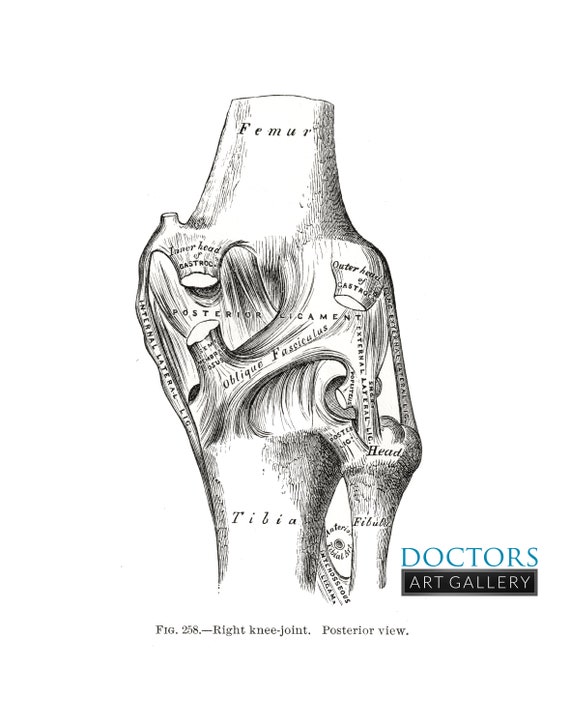This detailed black-and-white medical illustration presents a posterior view of a right knee joint, displayed against a pristine white backdrop. The top part of the image showcases the femur bone, meticulously labeled with both the inner head and outer head of gastro. Below the femur, the knee joint is richly annotated, identifying various ligaments such as the posterior ligaments, internal and external lateral ligaments, and the oblique fasciculus. The tibia and fibula bones are clearly marked towards the bottom of the diagram, with the surrounding details of muscle structures intricately illustrated. Every component is carefully labeled for educational purposes, affirming its utility in medical teaching materials. Prominently featured in the lower right corner, the brand name "Doctor's Art Gallery" appears in a combination of blue and gray capital letters. Beneath the figure, it reads "Figure 258, Right Knee Joint, Posterior View," encapsulating the precision and educational intent of this carefully rendered anatomical sketch.